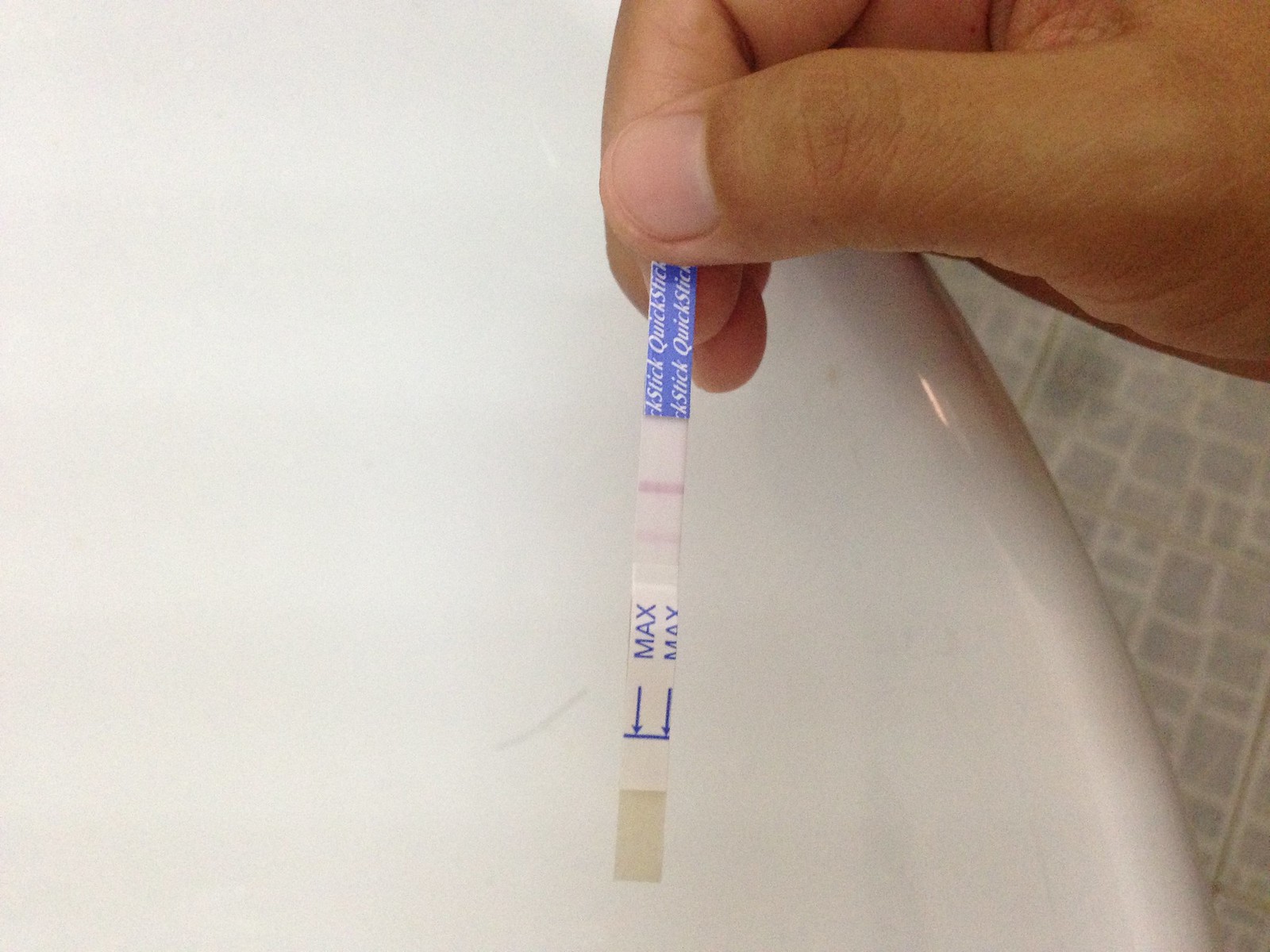In this horizontal image, a fair-skinned hand is depicted holding a quick stick test strip vertically at the center of the photograph. The visible parts of the hand include the thumb and the first two fingers, along with a segment of the palm between the thumb and the base of these fingers. Positioned in the upper right-hand corner of the frame, the hand firmly grips the top blue portion of the test strip.

The test strip extends downward, displaying a section with faintly colored lines, indicative of the test results. Beneath this, the test strip is marked with a demarcation indicating the maximum fluid level for testing. The backdrop consists of a porcelain sink, possibly almond or off-white in color, creating a neutral and clean environment for the focus on the test strip.